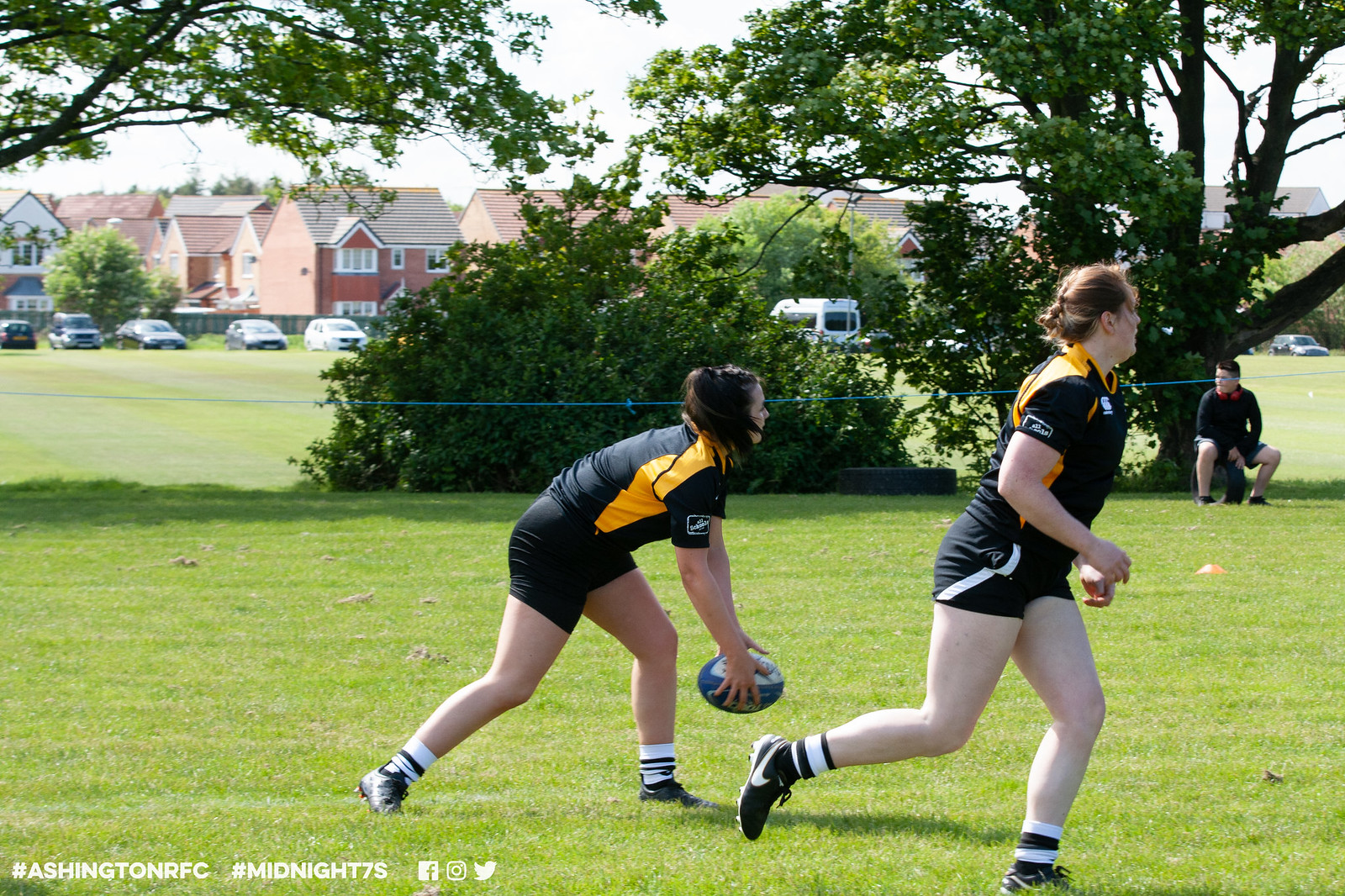The photograph captures a vibrant outdoor scene featuring two women playing rugby on a lush green field. Central to the image, one woman is gripping the rugby ball as her teammate runs alongside her. Both athletes are clad in black and yellow uniforms with small, barely readable lettering, and they wear black shoes. In the background, a person is seated, likely watching or refereeing the game. The setting is encompassed by green trees and a row of houses of varying colors, from white to red, creating a sense of community around the field. Notably, the scene takes place at Ashington Rugby Football Club, as suggested by the hashtags and social media symbols for Facebook, Instagram, and Twitter displayed at the bottom left corner. A blue rope delineates the edge of the playing area, subtly indicating the boundaries of the rugby field. Overall, the dynamic composition emphasizes the intensity and camaraderie of the game while situating it within a picturesque and supportive community environment.